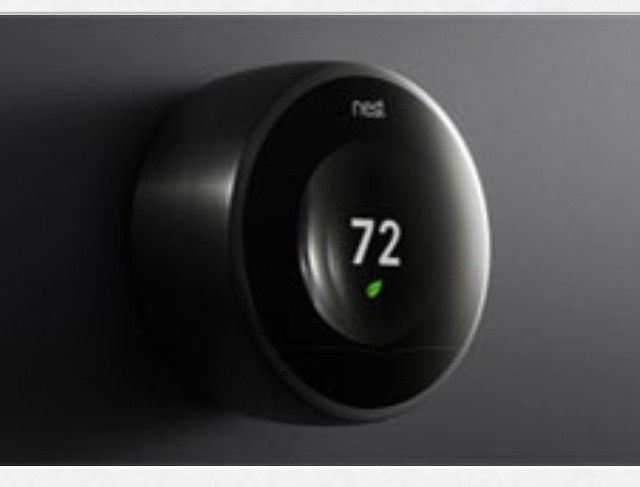The photograph captures a Nest thermostat prominently displayed on a dark gray wall. The lighting in the image creates a striking contrast, with the left side enveloped in deep shadow, while the right side, particularly the upper right-hand corner, is bathed in light. The thermostat is centrally placed and viewed from a slight angle, showcasing its sleek, round design. 

The body of the thermostat appears to be crafted from stainless steel, giving it a modern and sophisticated look. The device features a prominent black border around its circular face, which is primarily gray. At the top of the black border, the word "Nest" is inscribed in white. Dominating the center of the display is the number "72," also in white, indicating the current temperature setting. Just below the number "2," there is a small, green leaf icon, suggesting energy efficiency or eco-friendliness. The overall composition of the photograph emphasizes the thermostat's elegant design and functionality against the backdrop of the nuanced wall.